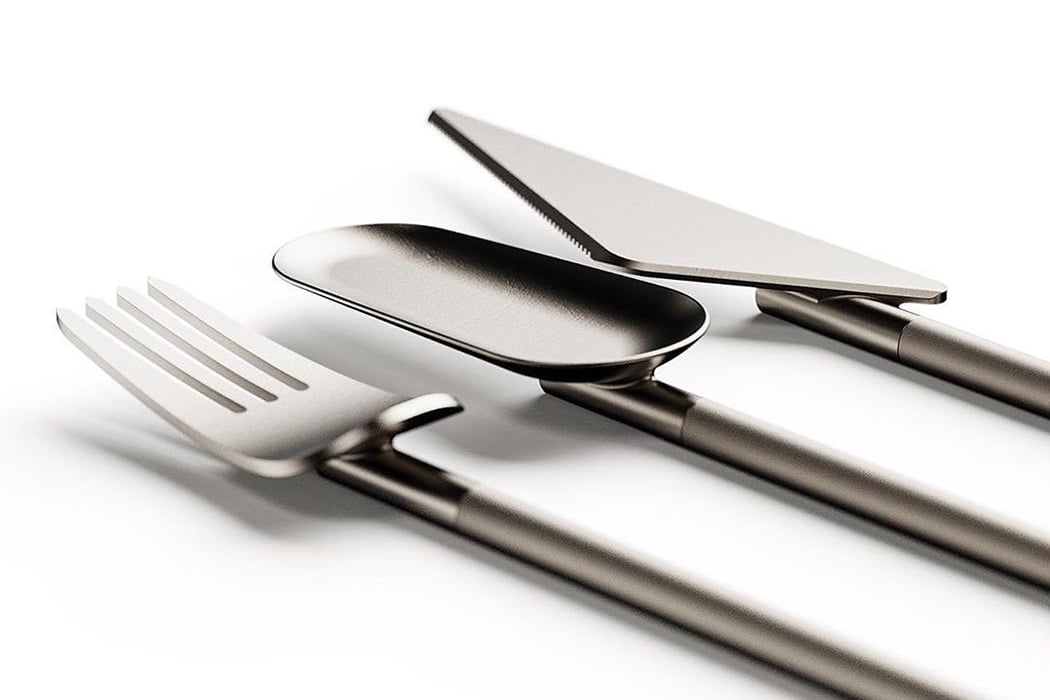The close-up image depicts three pieces of modern, artistic cutlery arranged at an angle on a white surface, casting subtle shadows. The set includes a fork on the left, a spoon in the center, and a knife on the right. All pieces are primarily metallic, though the handles appear to be made of acrylic or a similar transparent material, giving them a contemporary look.

The fork has a thin, cylindrical handle and a distinctive design where the pronged end scoops upward, appearing somewhat detached from the handle. The spoon in the center has an unconventional structure, with the oval, scoop-like bowl mounted atop the handle, resembling a small measuring cup. Lastly, the knife on the right features a flat, triangular blade with the cutting edge on one of the shorter sides, and both the remaining short side and the long side are smooth. The innovative designs lend a modern and somewhat experimental aesthetic to the set.